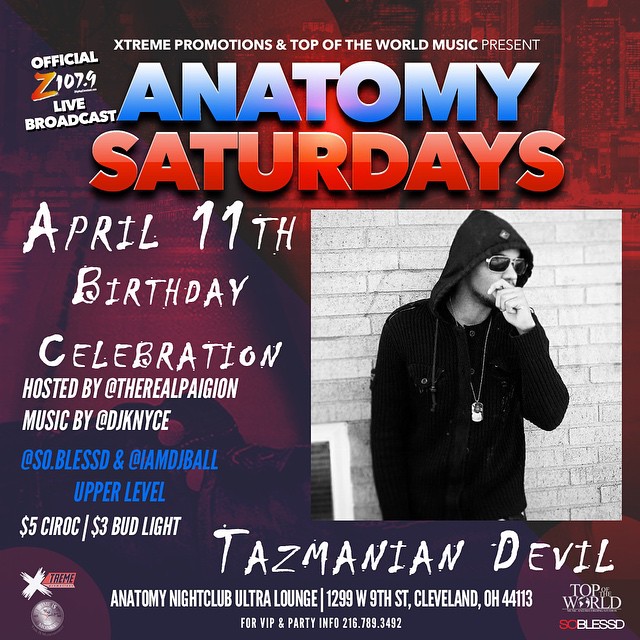The flyer for a nightclub event features a dark brick red and maroon color scheme with a blurred column background. At the top, it reads in white text, "Extreme Promotions and Top of the World Music Present," followed by "ANATOMY" in bright blue all caps and "SATURDAYS" in bright red all caps. The left-hand side includes the logo for "Official Z 107.9 Live Broadcast." 

In a handwritten white font, the flyer announces "April 11th Birthday Celebration hosted by @TheRealPagan, music by @DJKNYCE." Below this, in blue text, it adds "@SoBlessed and @IAmDJBall." The upper level entry fee is "$5" with "$3 Bud Light" and "CIROC" specials.

To the right-hand side, there is a black and white photo of a man in a black hoodie with the hood up, wearing dark sunglasses, and holding his hand in a fist near his mouth. He is also sporting a necklace and leaning against a light brick-colored building. Below this image, in big white print, it says "Tasmanian Devil."

Further details at the bottom in white text provide the address: "Anatomy Nightclub Ultra Lounge, 1299 West 9th Street, Cleveland, Ohio 44113," and a contact number for VIP and party info: "216-789-3492." The lower right corner has logos for "Top of the World" with an earth symbol in the 'O,' "SO BLESSED" in red and white text, and "XTREME," with 'X' in white and 'TREME' in black against a red rectangle.